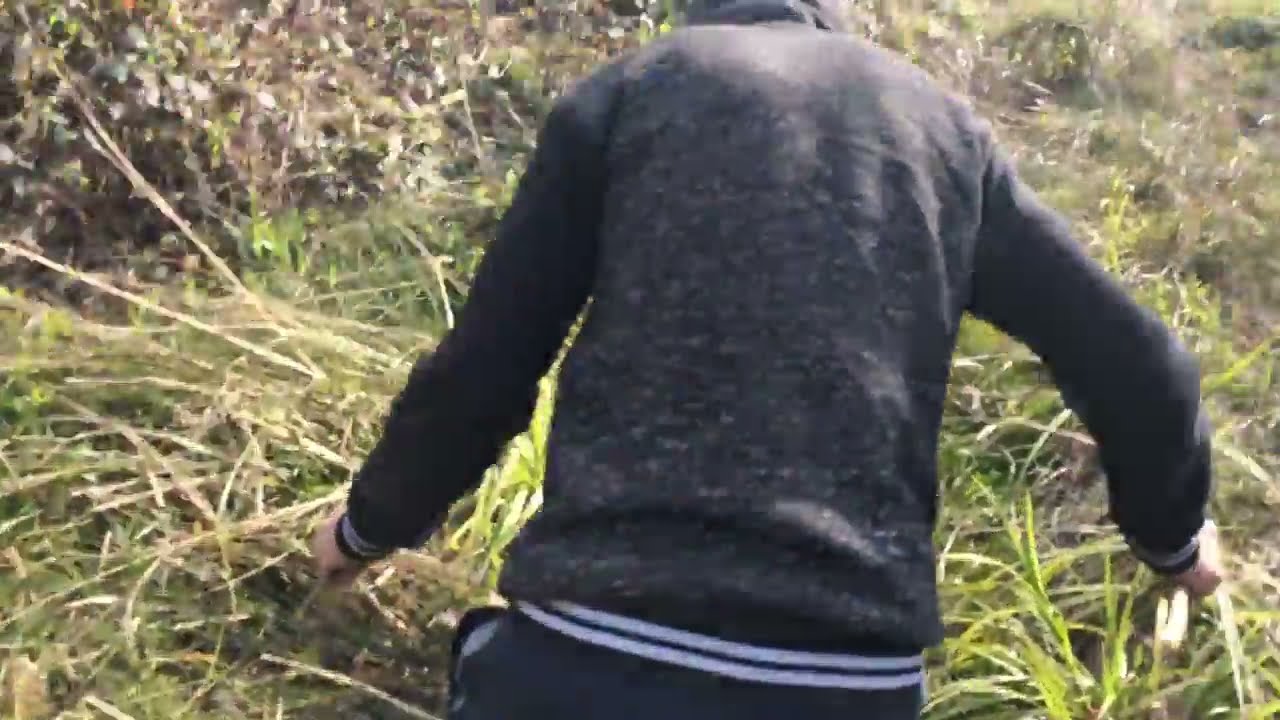In this daytime outdoor image, the camera captures a downward angle view of a person standing in a field of long, green and yellowish grass, possibly mixed with hay and clover. The grass appears smushed and stepped on, indicating the person has been walking through it. The person is visible from the mid-back down, wearing a black and white jacket with a pinstripe around the waist and tight black pants with a pocket on the right side. Their footwear consists of black shoes with two white stripes. The focus on the lower half of the person's body, including their rear end and legs, suggests the photo might have been taken accidentally, potentially while the camera was held in hand. The scene is simple yet detailed, highlighting the interplay of natural elements and casual attire.